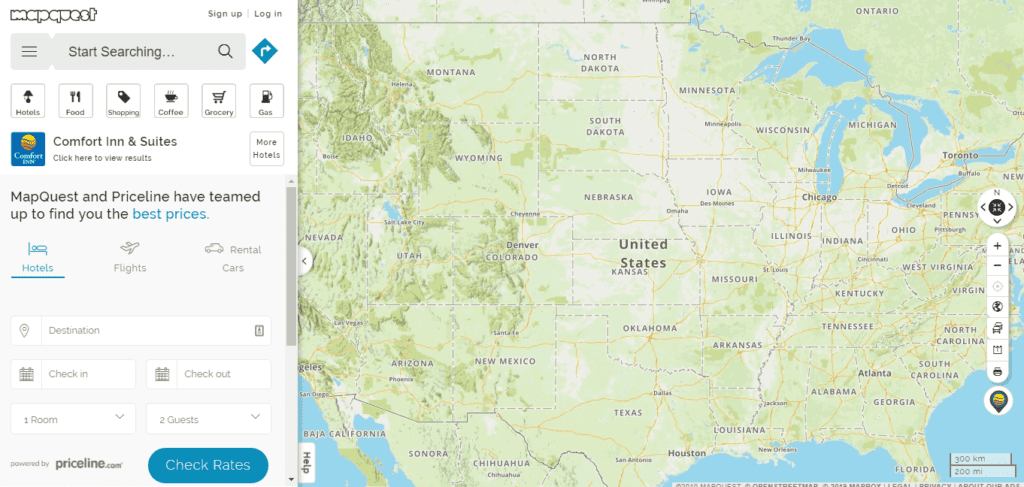The image displays a screenshot of MapQuest's user interface. On the left-hand side, there is a vertical section featuring the MapQuest logo prominently at the top left with its letters outlined. Directly below the logo is a 'Start Searching' search bar, inviting users to input their queries. To the upper right of this section are convenient 'Sign Up' and 'Log In' buttons for user access.

Beneath the main search bar, there are six horizontally aligned icons labeled as follows: 'Hotels,' 'Food,' 'Shopping,' 'Coffee,' 'Grocery,' and 'Gas,' each representing a category of services that can be searched for. Under this row of options, there is a banner promoting 'Comfort and Suites' with a call-to-action reading, "Click here to view results," and to the right, it mentions additional options with "More hotels."

Further down, an informational note indicates that "MapQuest and Priceline have teamed up to find you the best prices." Below this message, three tabs can be seen, each corresponding to a different type of booking service: 'Hotels,' 'Flights,' and 'Rental Cars.'

The right-hand side of the image features a map of the United States, providing a geographical interface for navigation and location searches.